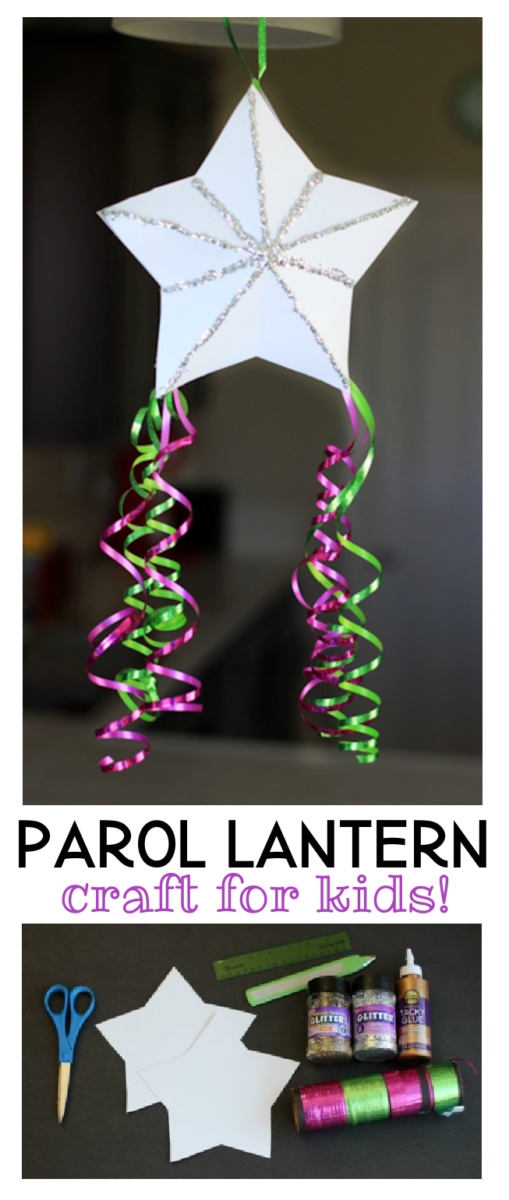The advertisement features an engaging craft activity for kids called the "Parol Lantern Craft." It's presented within a long vertical rectangle. The upper two-thirds of the advertisement showcase a detailed photograph of a festive five-pointed star made from paper. This star is intricately adorned with silver glitter in radiating patterns from the center to the points, creating a shimmering effect. From the bottom two points of the star hang colorful streamers—purple and green—that add a playful touch to the decoration.

Below this captivating image, bold text reads "Parol Lantern Craft for Kids!" highlighted in blue, making it cheerful and appealing. Near the bottom of the advertisement, there is a smaller photograph displaying all the necessary materials to create the craft. These include two paper stars, rolls of pink and green ribbon, jars of glitter, a tube of glue, a ruler, a pair of scissors, and several markers. The clear layout of materials helps in guiding kids and parents alike to prepare for this fun and creative project.